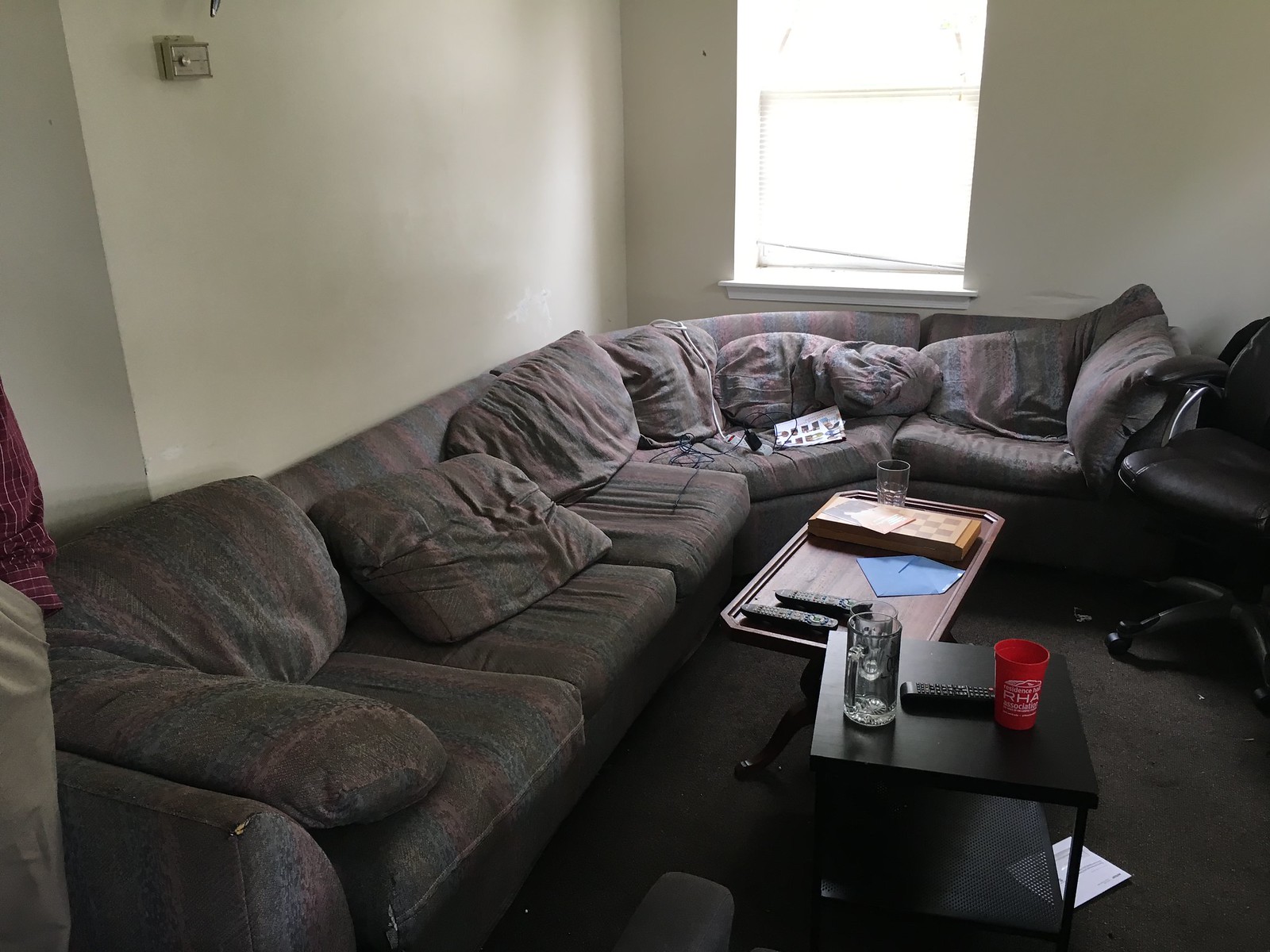The image depicts a corner of a somewhat cluttered and well-used living room inside an apartment. Dominating the room is a sizeable gray corner couch with red accents, which appears worn and untidy, with cushions displaced and covers crumpled. Various objects, including some cables, are strewn across the couch. Near the couch are two small tables: a shorter brown wooden table and a slightly taller black table. On the wooden table rests a clear glass and two black TV remote controls, while the black table holds a red cup, another clear glass, a beer stein, and another black remote control. The room is brightly lit by sunlight streaming through an unadorned window. The walls are painted white, featuring an air conditioning control unit in the upper left corner. In the distance, a black rocking chair is barely visible. Additionally, a man dressed in khaki pants and a red shirt is seated at the end of the couch. The apartment floor is dark gray, contributing to the overall impression of a lived-in but currently untidy space.